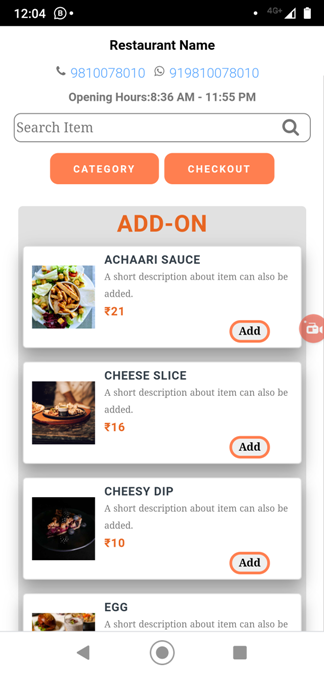A detailed screenshot of a food ordering app interface on a smartphone, likely in India, with timestamps, connectivity indicators, and more. The image reveals the screen at 12:04 PM, displaying crucial details such as the battery life and network signal strength.

At the top of the app interface, the restaurant's name is prominently displayed, accompanied by two contact numbers—one for direct phone calls and another for WhatsApp, indicated by a recognizable icon. The operating hours of the establishment, running from 8:36 AM to 11:55 PM, are clearly listed below the contact information.

A functional search bar is positioned beneath these details, enabling users to enter specific food items they are looking for. Just below the search bar are two interactive buttons labeled "Category" and "Checkout," aiding in seamless navigation and order processing.

The current section of the app is focused on "add-ons," allowing users to enhance their meals with extra items. The first item presented is "Achari Sauce," pictured on a plate that appears to include sticks resembling french fries and vegetables. Beneath the image is a placeholder for a short description, indicating this might be a developer version or mock-up of the app.

Following the achari sauce, there are images and titles for additional add-ons: a cheese slice, a cheesy dip, and an egg. Each item photo is accompanied by a placeholder text stating, "A short description about item can also be added," further suggesting that this app version is under development or testing.

The product prices are listed in Indian Rupees (₹), confirming the app's non-USA origin. The overall interface design and structure hint at its user-friendly functionality, though the incomplete item descriptions suggest it is still in the refinement stages.